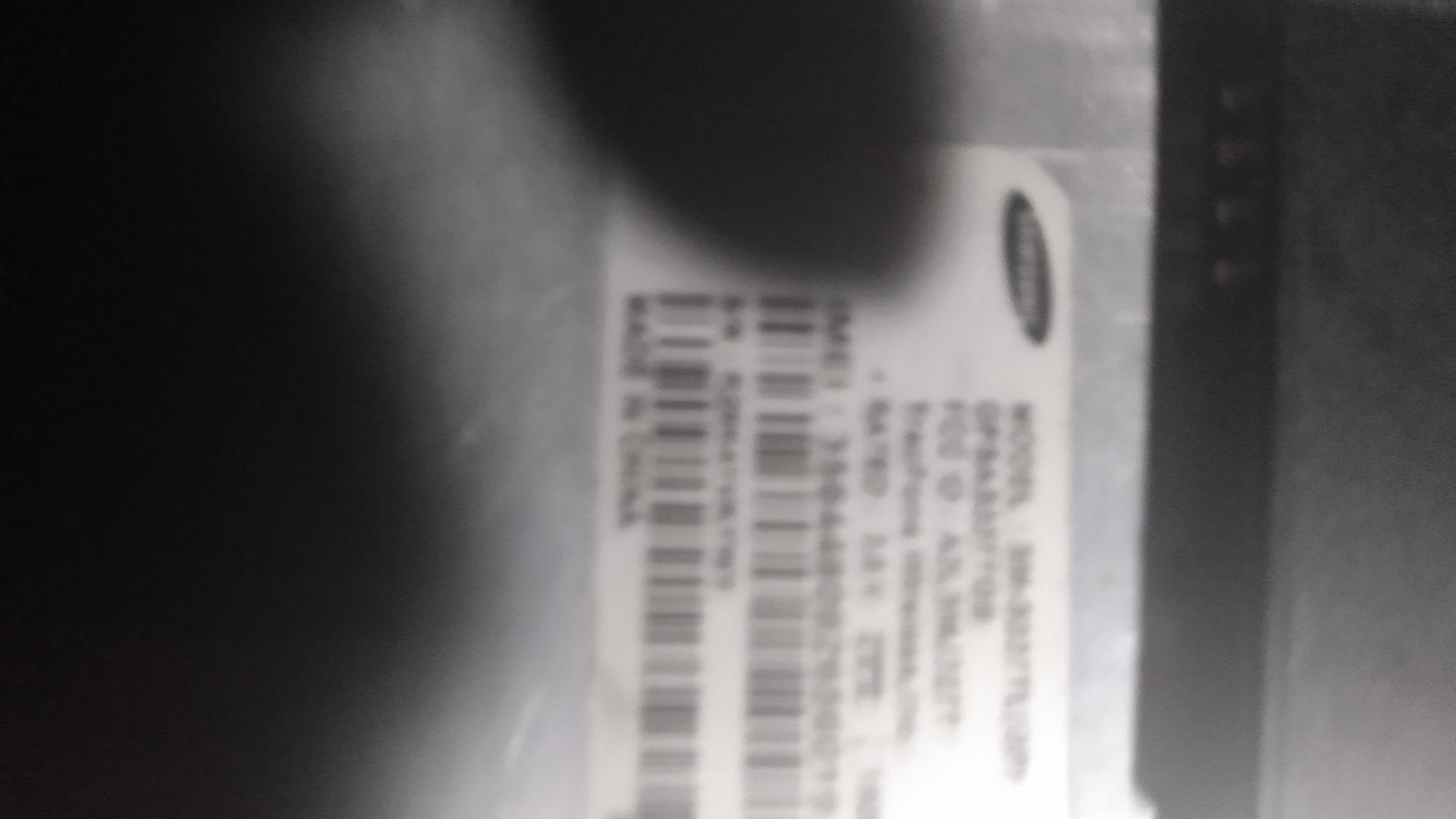This rectangular, low-resolution photograph appears shadowy and heavily blurred. On the right side, a darkened area occupies roughly one-fifth of the image's vertical length. Adjacent to this, the scene lightens to a gray hue accentuated by scattered white specks. A vertically oriented label in this lighter zone extends from the top to the bottom. The label is white with black text and features two narrow scan code bars running vertically. However, the details of the text and numbers on the label are indiscernible. To the left of the label, the image continues in a grayish-white shade that transitions into progressively darker tones, culminating in a black section along the photograph's left edge.